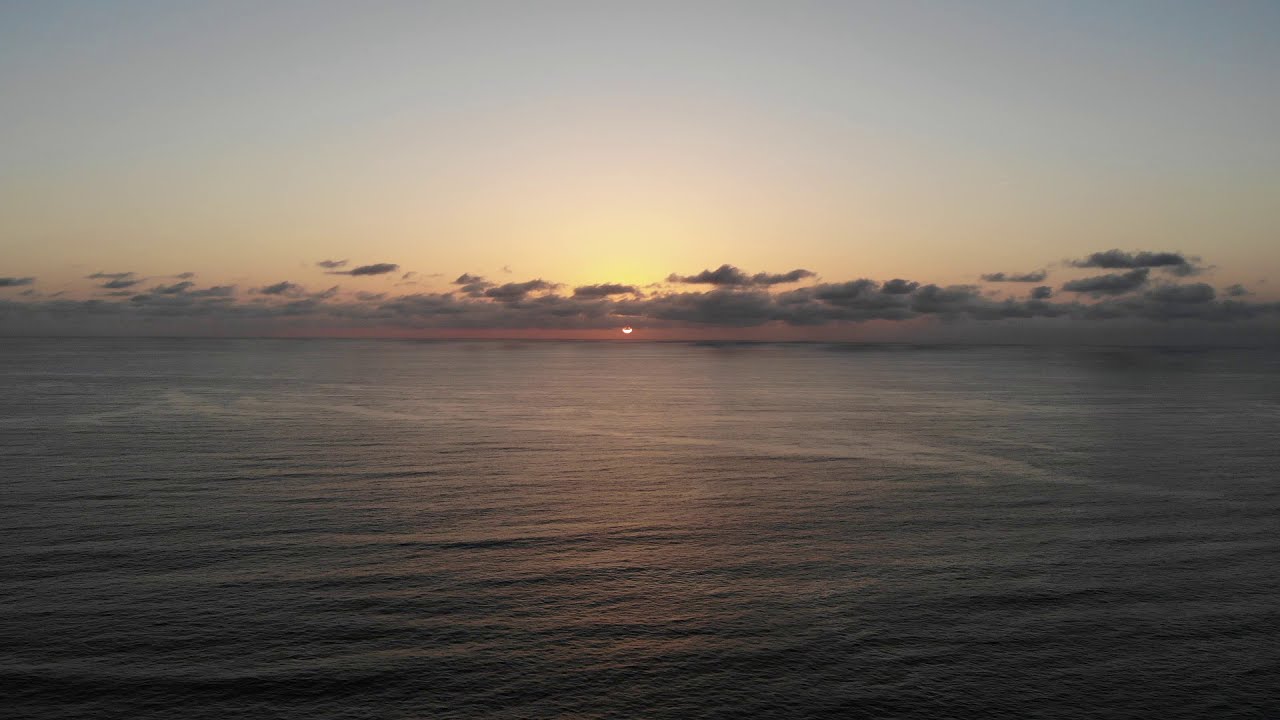The image captures a serene ocean sunset. The horizon is filled with scattery grey and black clouds forming a straight line from left to right, obscuring parts of the red sun that is peeking out. The water is mostly calm, with slight ripples, appearing extremely dark and blending with the shadows cast by the retreating light. The golden sunlight bounces off the ocean’s surface, though the water remains inscrutable, revealing no reflections. Above the horizon, the sky transitions in a stunning gradient from blue at the top, through yellow and orange, to a deep red closest to the water. The atmospheric hues also intermingle with touches of purple, adding to the visual appeal of the scene. The sun, nestled amidst these colors, provides a striking focal point, illuminating the layered hues and tranquil water below.